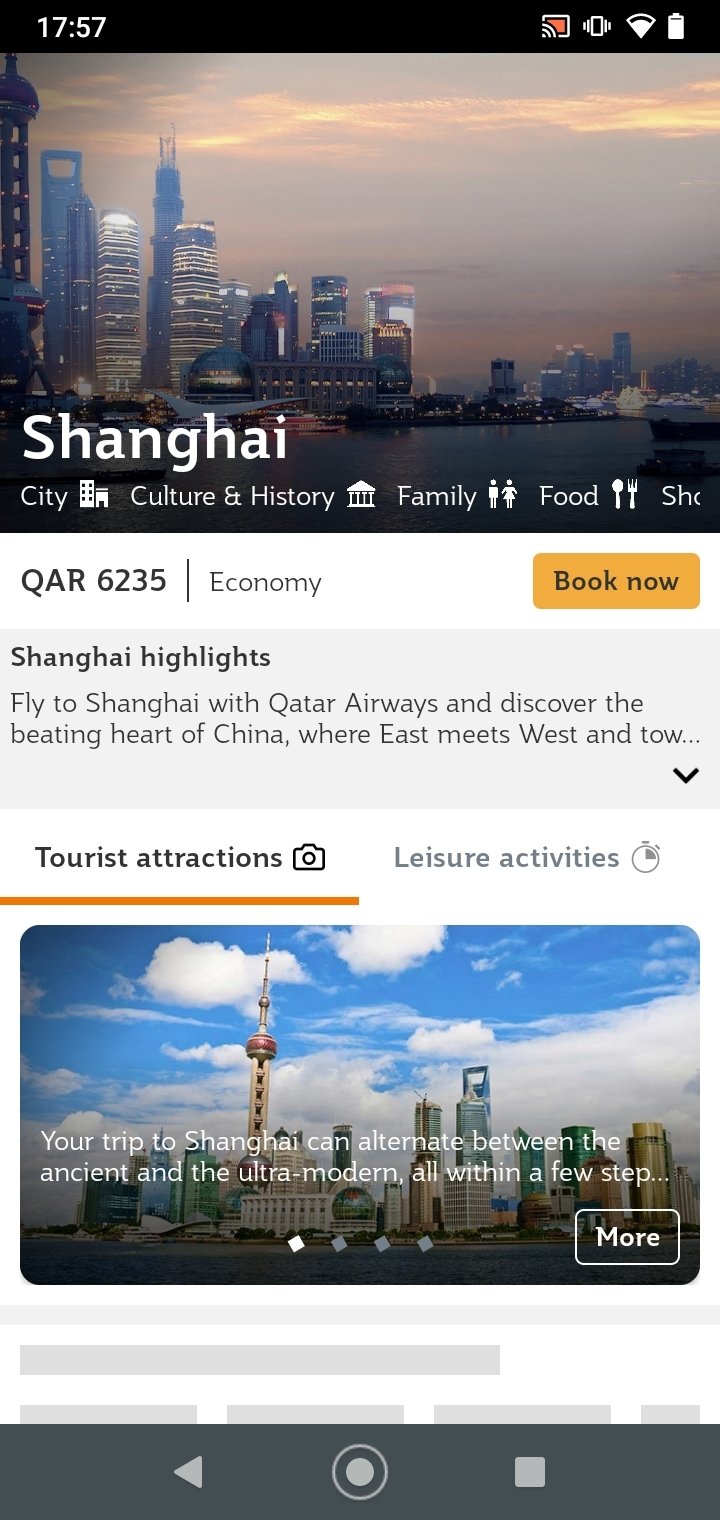Captured from an Android device, the screenshot appears to show a detailed informational interface about Shanghai. The top bar of the screen, on the left, displays the time in military format, reading 17:57. On the right side, there is a series of icons: a red "RS" light in a square, a phone signal icon next to it, a nearly full Wi-Fi signal, and a mostly full battery indicator.

Beneath this, a vibrant image of Shanghai is prominently featured. Underneath the image, the screen lists various categories relevant to Shanghai, each accompanied by a corresponding icon: "City," "Culture and History," "Family," and "Food," the latter represented by a fork and spoon icon. Partially cut off text can be seen, starting with "SH."

Further down on the screen, the text "QAR6235" is visible, followed by the word "Economy." To the right, an orange "Book Now" button prompts action. Below this section, set against a gray background, is the heading "Shanghai Highlights," accompanied by a drop-down arrow. Underlined in orange is the phrase "Tourist Attraction," next to a camera icon, followed by "Leisure Activities."

Another image of Shanghai appears at the bottom, with navigation indicators showing three little dots and one highlighted dot, implying a carousel of images or options. A "More" button is situated next to these indicators, inviting further exploration.